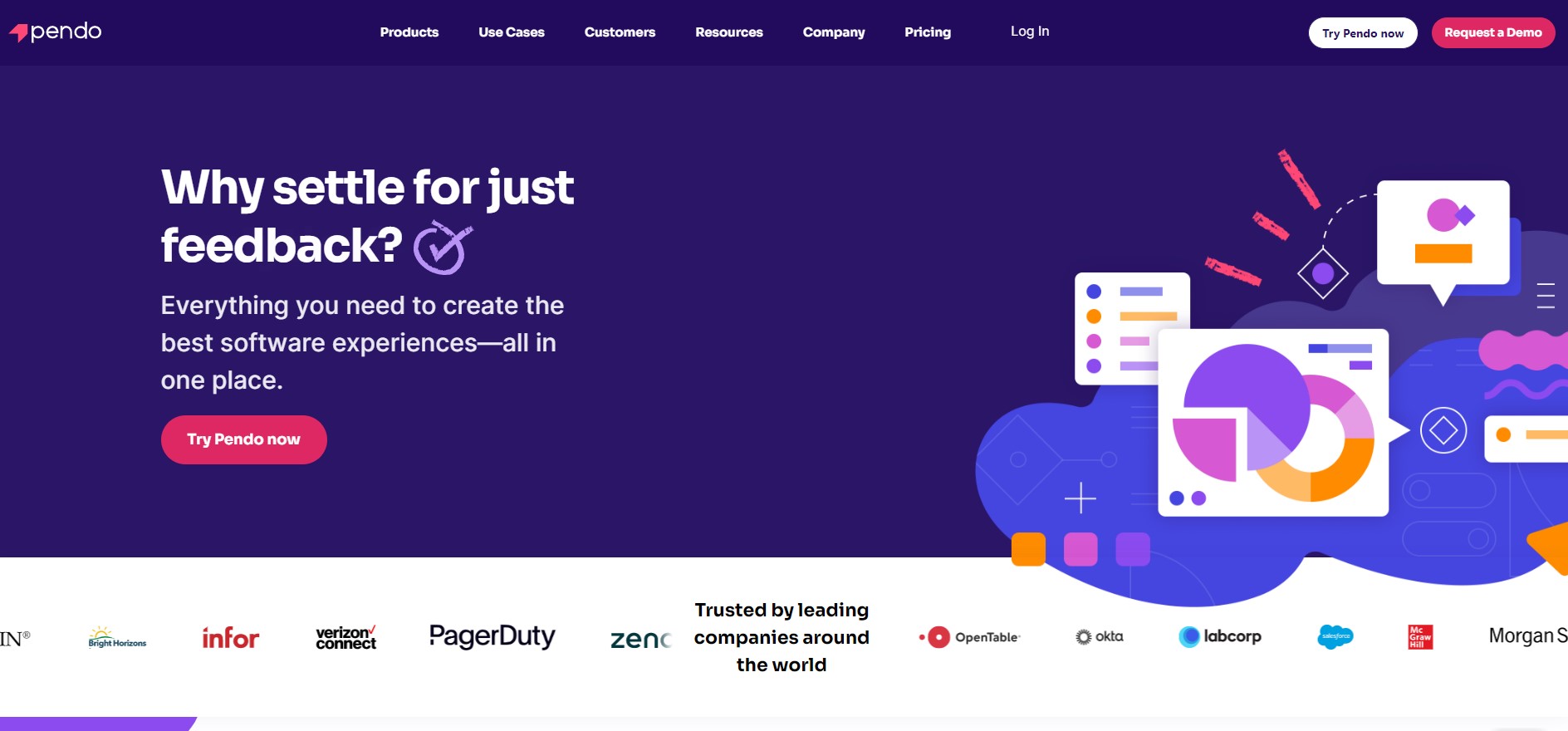The image depicts a webpage from Pendo, showcasing a user-friendly interface with a purple and white color scheme. At the top of the page, the Pendo logo is prominently displayed alongside a navigation menu with categories: Products, Use Cases, Customers, Resources, Company, Pricing, and Login. Additionally, there are conspicuous buttons labeled "Try Pendo Now" and "Request a Demo."

Beneath the navigation, a compelling headline reads, "Why Settle for Just Feedback? Everything you need to create the best software experience is all in one place. Try Pendo Now." This is followed by an array of icons representing notable companies such as Bright Horizons, Infor, Verizon Connect, and PagerDuty, illustrating that Pendo is "Trusted by leading companies around the world." Other companies listed include OpenTable, LabCorp, Salesforce, McGraw-Hill, and Morgan S.

The main body of the page features a graphic consisting of circular shapes, charts, and data representations typically found in a software environment, emphasizing the comprehensive analytical tools Pendo offers. The overall aesthetic highlights Pendo's extensive suite of software solutions, visually reinforcing their modern and robust approach to improving software experiences.